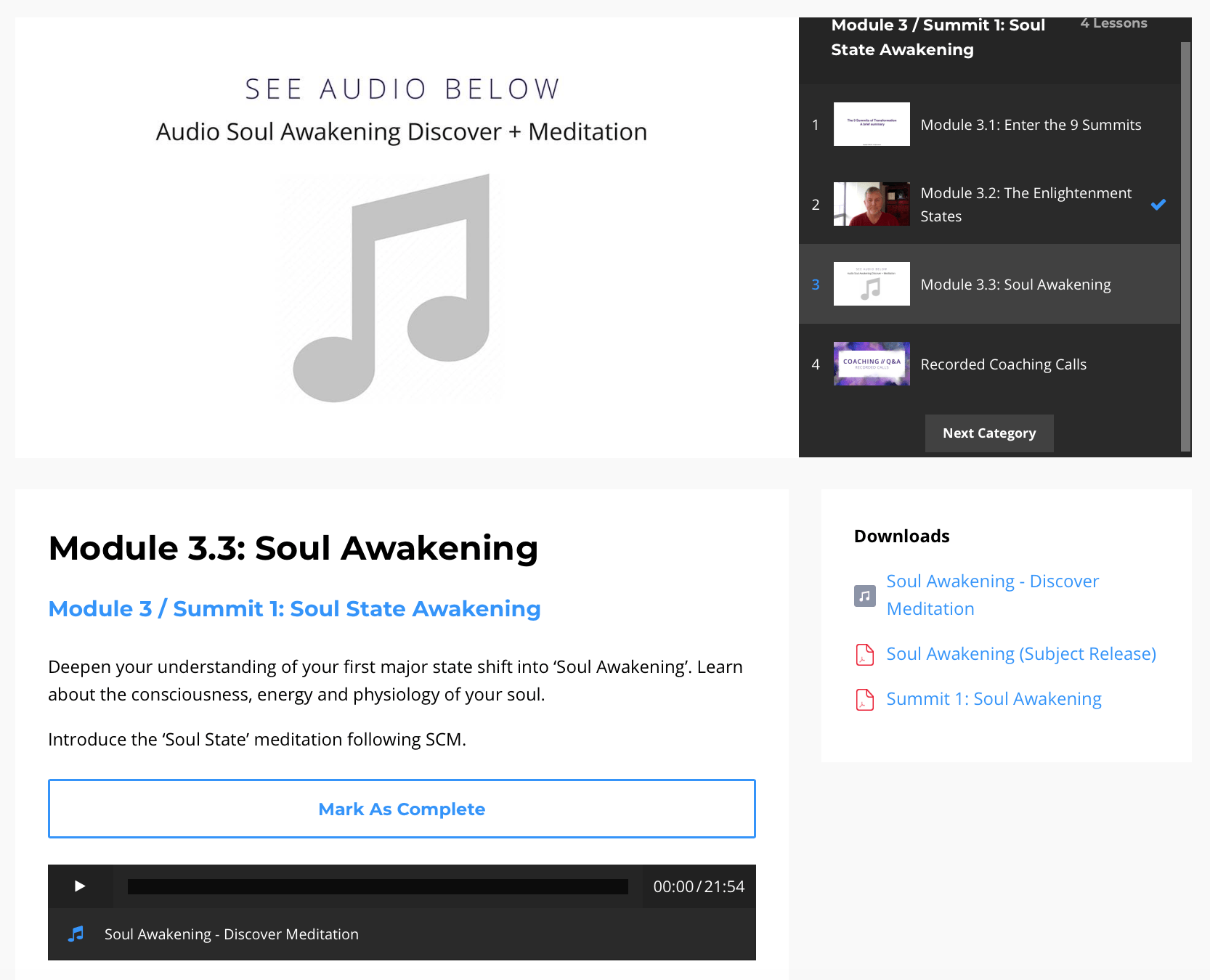The image depicts a music-themed website layout, divided into two primary sections: the left and the right. The left section is dominated by a prominent white square that spans a significant portion of the area. Within this white square, the heading "See Audio Below" is followed by the titles "Audio Soul Awakening" and "Discover Plus Meditation." 

Centered within this block is an oversized musical note icon, which draws immediate attention. Below this icon, there is a smaller block labeled "Module 3.3: Soul Awakening." Further down, it reads "Module 3 / Summit 1: Soul State Awakening." 

Accompanying these titles are descriptive sentences aimed at encouraging deeper understanding and engagement: "Deepen your understanding of your first major state, shift into soul awakening. Learn about the consciousness, energy, and psychophysiology of your soul."

At the bottom of the section, there is an actionable button labeled "Mark as Complete," suggesting that users can track their progress through the modules.